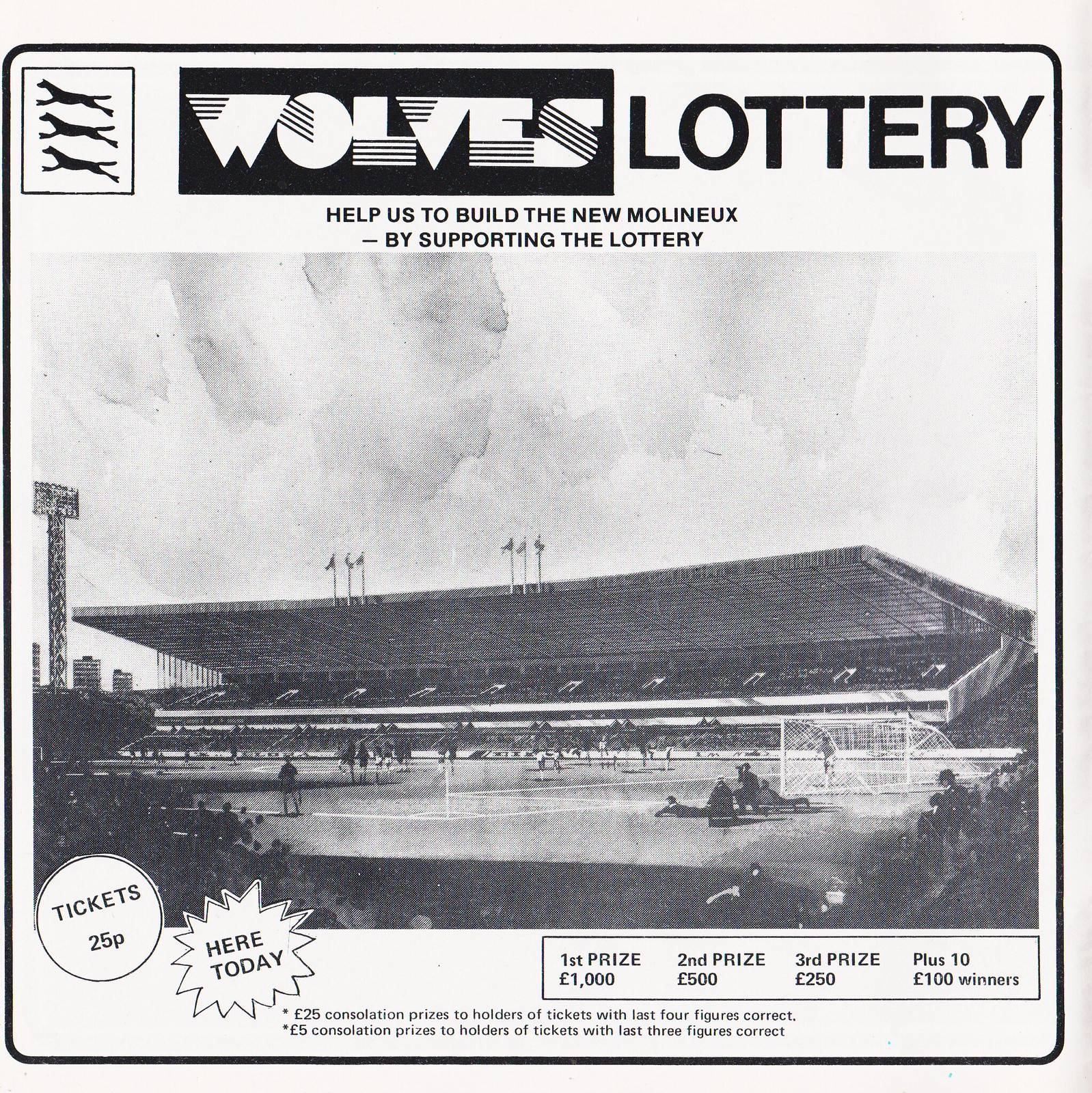The image appears to be an old black-and-white advertisement for a lottery, possibly from a magazine or newspaper, set on a white piece of paper with a thin, black rounded-border creating a square shape with beveled edges all the way around. At the top inside of the black line, there’s a light gray header featuring a black square on the left with an image of three flying wolves or cheetahs. To the right, there is a black rectangle with white text that reads "Wolves" and next to it, larger black text saying "Lottery". Below this header, the text states: "Help us to build the new Molyneux by supporting the lottery". The main portion of the image showcases an artist's black and white rendition of a large grandstand, potentially part of a football pitch, with an awning over raised bleachers and several people depicted in the scene. At the bottom left, there is a white circle with a black outline stating "Tickets, 25p." To its right, a jagged star reads "Here today." Further right, another square with a black outline details the lottery prizes: "First prize, 1,000 pounds. Second prize, 500 pounds. Third prize, 250 pounds. Plus 10, 100-pound winners." At the bottom, additional text specifies: "25-pound consolation prizes to holders of tickets with the last four figures correct. Five-pound consolation prizes to holders of tickets with the last three figures correct." Some legal text is also included at the bottom.